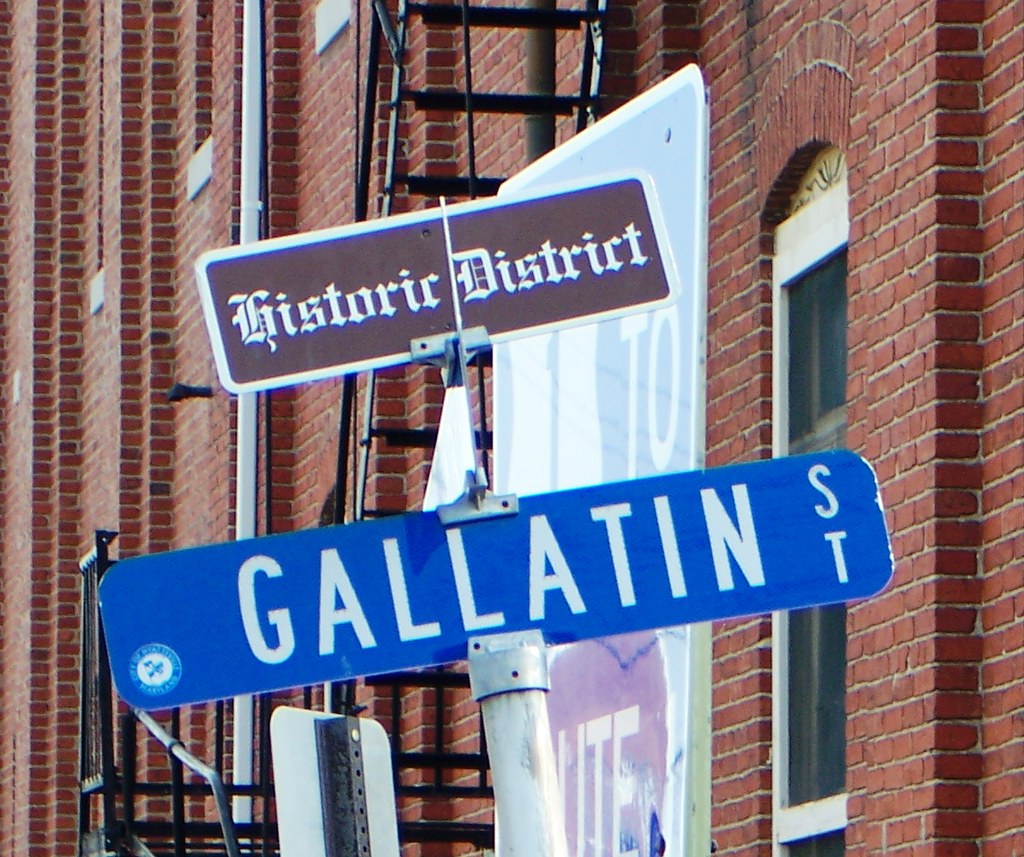The image captures a bustling downtown scene centered around a prominent street sign pole with two signs at the top. The top sign features a brown background with white lettering that says "Historic District" in an old-fashioned font. Below it, a blue sign with white lettering marks "Gallatin Street," complete with a white insignia in the bottom left corner. 

In the background, a tall red brick building stretches into the sky. This building showcases several arched windows with white frames and black interiors, one of which prominently displays a partially visible white flag bearing the word "2" and the word "light" set against a purplish background with hints of green on the right. Clinging to the side of the building, a black iron fire escape zigzags upwards.

Adding to the urban ambiance, near the center-left of the image, the back of another street sign is partially visible, characterized by its black rear and white front. Overall, the scene is rich with architectural details and signage, highlighting the storied charm of this downtown historic district.